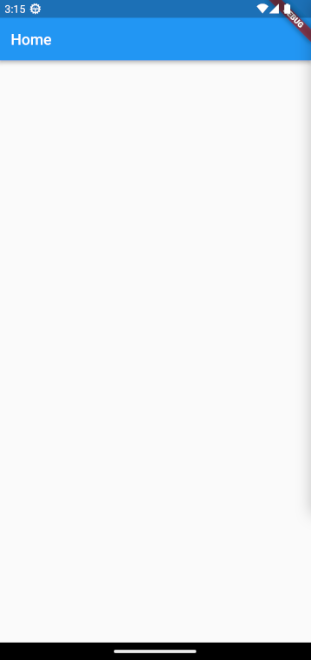This image is a vertical screenshot from a mobile or smartphone interface. The screen is largely blank and white, framed by various banners and icons. At the very top, there is a thin, dark blue strip featuring the time "3:15" in white text, and an icon that is white with a blue center on the left side. The right side of this strip includes a battery icon and two other unidentified icons. A red diagonal banner labeled "BUG" is positioned in the top right corner of the image.

Beneath the darker blue strip, a wider, lighter blue banner runs across the screen, displaying the word "Home" in white text, indicating that this is the user’s home page. 

At the very bottom of the image, there is a thin black banner with a thin white horizontal line running across the center. Additionally, the right edge of the screen, from the top of the white section down to about three-quarters of the way, features a subtle, lighter gray border, almost blending into the white background. 

The overall appearance of the home page is blank, with no icons or apps visible, giving it a minimalist look.